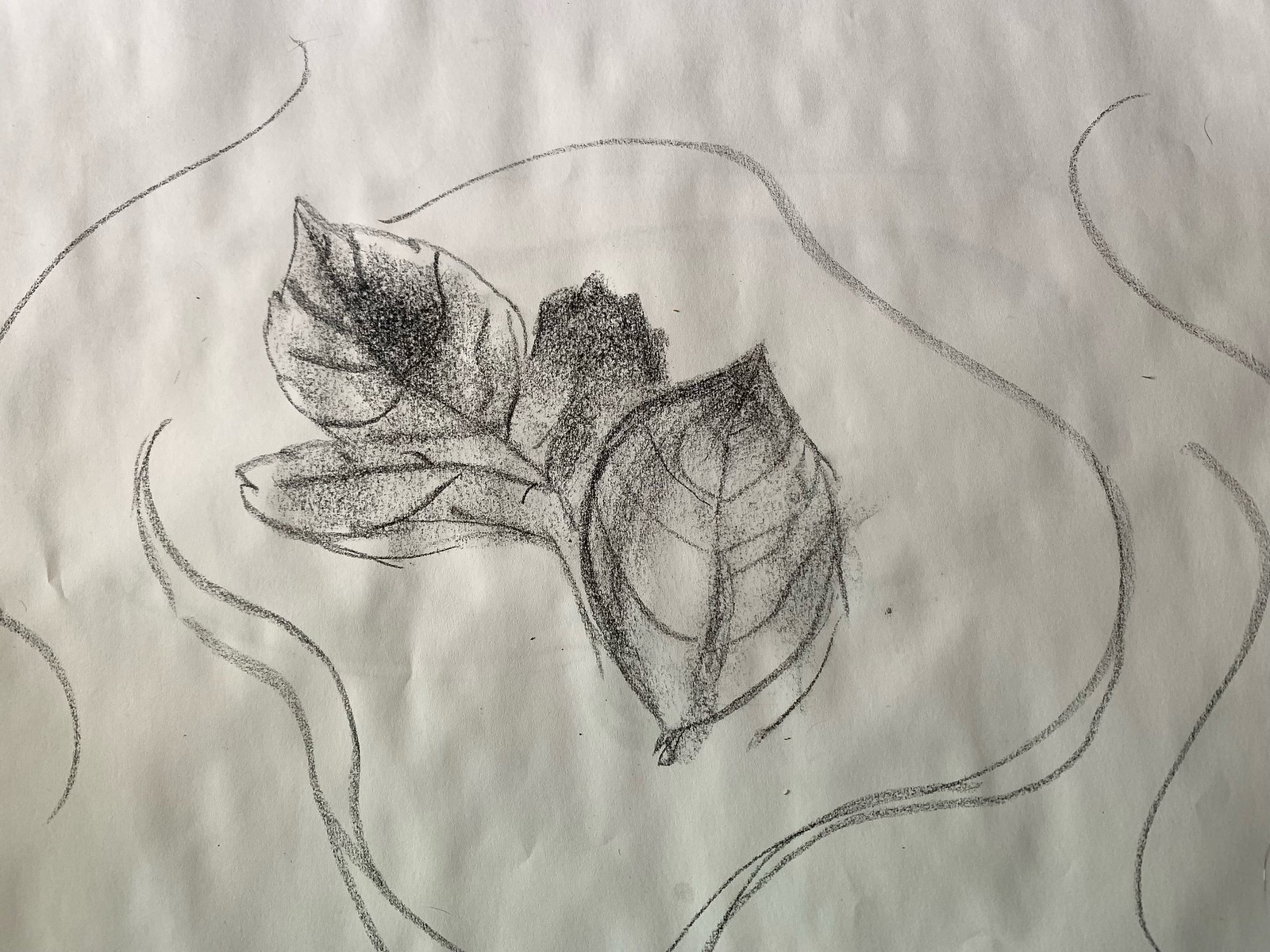This detailed photograph captures an intricate illustration rendered on a clean, white sheet of paper. Central to the composition is a cluster of leaves, meticulously drawn to depict one prominently detailed single leaf in the foreground. Behind this, there are three additional leaves attached to a small branch, each exhibiting nuanced shading and texture suggestive of the medium used, likely charcoal or a soft graphite pencil. Surrounding this botanical ensemble are a series of flowing and dynamic squiggly lines, expertly designed to evoke the ethereal movement of smoke or delicate wisps of air, adding a whimsical and animated quality to the scene. The stark contrast between the black of the drawing and the pristine white background amplifies the artwork's striking details and the fluid elegance of the lines.